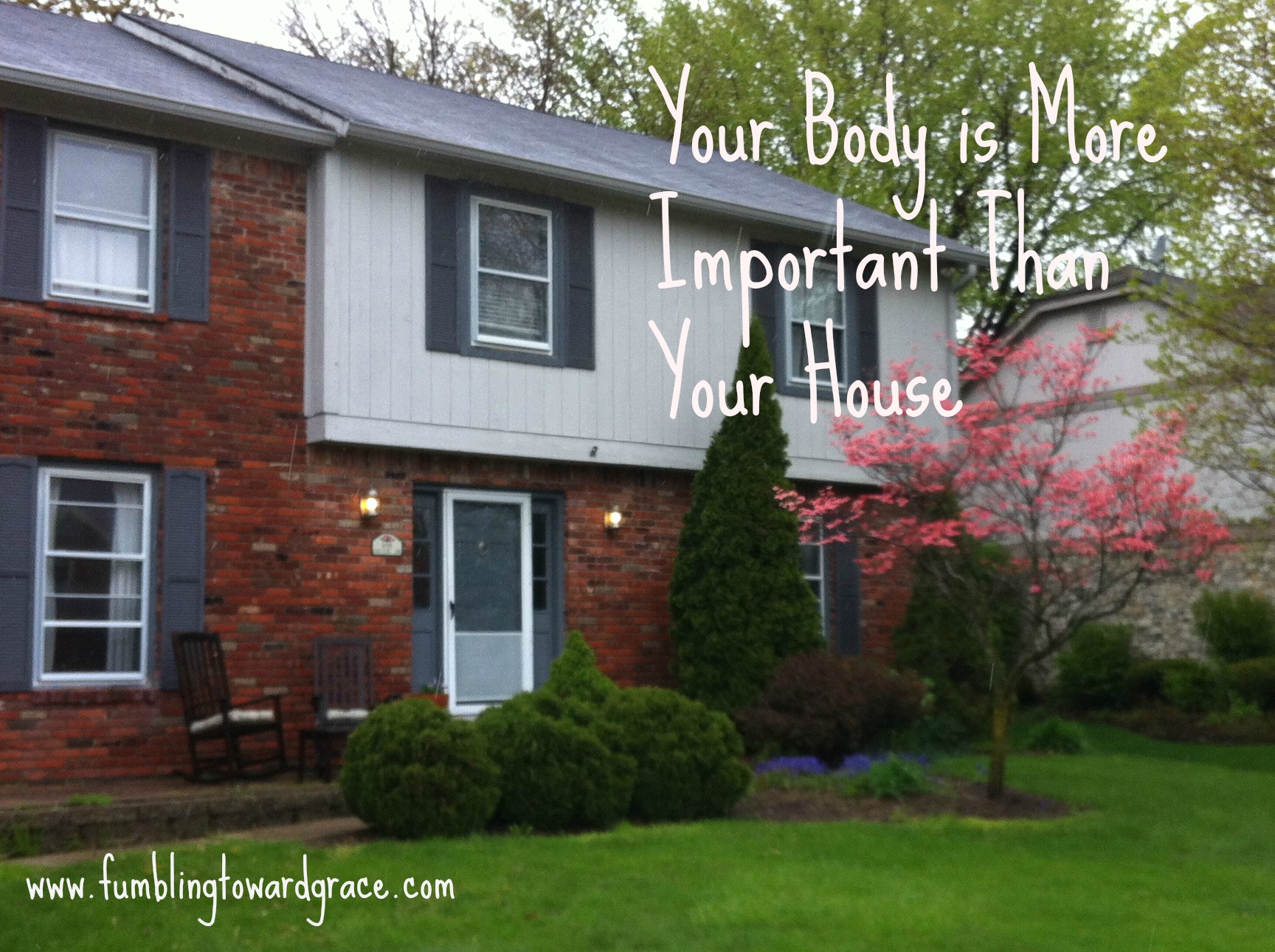The image depicts a charming two-story brick house, predominantly red brick with sections of white siding on the upper floor. The blueish-gray roof rises against a gray sky. The windows, framed with white trim and blueish-gray shutters, punctuate the building's facade. In the foreground, a well-manicured, expansive green lawn is bordered by neatly trimmed bushes. Prominently, a tall tree with pink blossoms stands to the right of the house, adding a splash of color to the scene. In front of the house, two brown chairs sit welcomingly by the single front door. To the right of the house, another building with white siding is partially visible, further framed by additional tall trees. Superimposed white text at the top of the image reads, "Your body is more important than your house," and the bottom left corner of the image includes the website address www.fumblingtowardgrace.com.